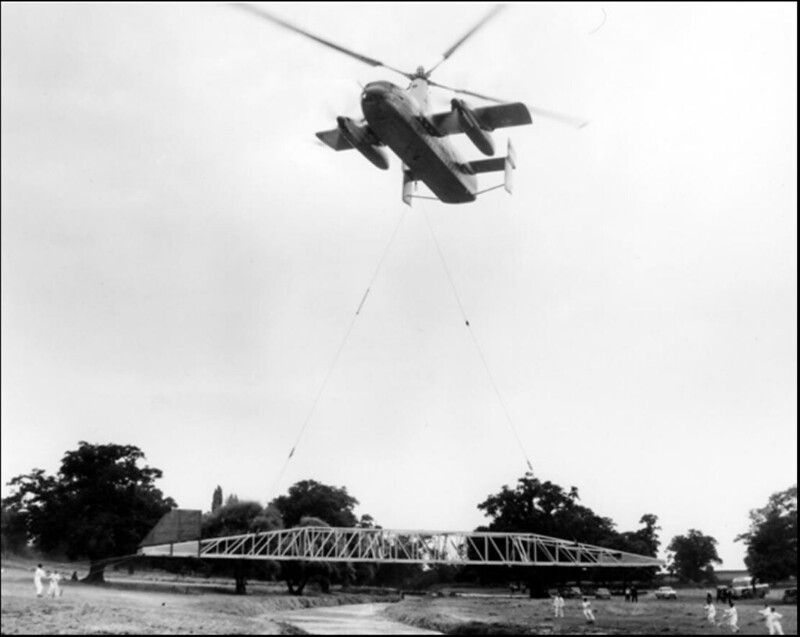A vintage black-and-white photograph depicts a substantial, old-fashioned helicopter-airplane hybrid in mid-air. This unique aircraft, appearing robust like a military cargo helicopter, features four large, plane-like wings, enhancing its intriguing hybrid design. Suspended from the helicopter by cables is a small, cage-like bridge structure, suggesting it might be part of a crane. The scene captures the helicopter delicately positioning the bridge over a small river. In the foreground, on the grassy field beneath the hovering aircraft, a crowd of people dressed in white can be seen observing the operation. These individuals, dwarfed by the imposing machine, are set against a backdrop of dark, dense trees under a clear sky, accentuating the vintage essence of the entire image.